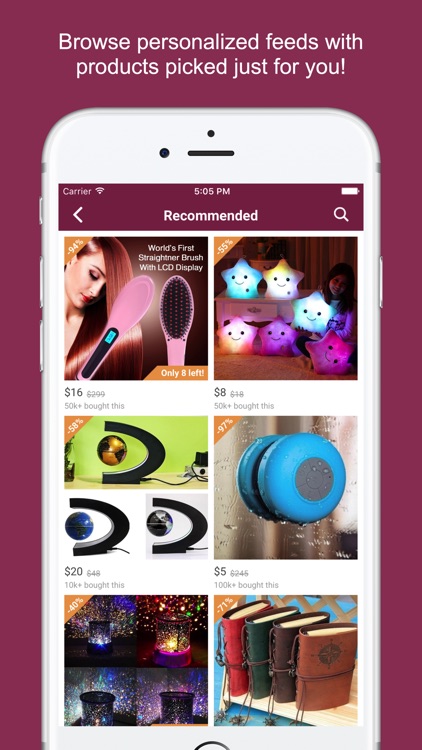A detailed screenshot showcases a section of a website, prominently featuring a promotional message at the top: "Browse personalized feeds with products picked just for you," in bright white text. This message is set against a dark purple background that envelops the top, left, and right sides of the screen.

Dominating the center of the image is a design of a cell phone with distinct white borders. At the top section of this phone interface, several elements are arranged: a "Recommended" tab centrally placed, a search bar to its right, a battery icon positioned above the search bar, the current time displayed in the middle, and a Wi-Fi connection icon on the left side, accompanied by a back arrow to its left.

Below this header, the main content is divided into six square images, each showcasing different products up for sale. Notably visible are the prices for the first four items, which are marked at $16, $8, $20, and $5 respectively. The remaining two products do not display their prices. The top four products also indicate discounts, highlighted by orange tabs on the top left of each image with white text specifying the percentage off.

Towards the bottom of the cell phone design, a small portion of the home button is subtly visible, rounding out the comprehensive layout of this screenshot.